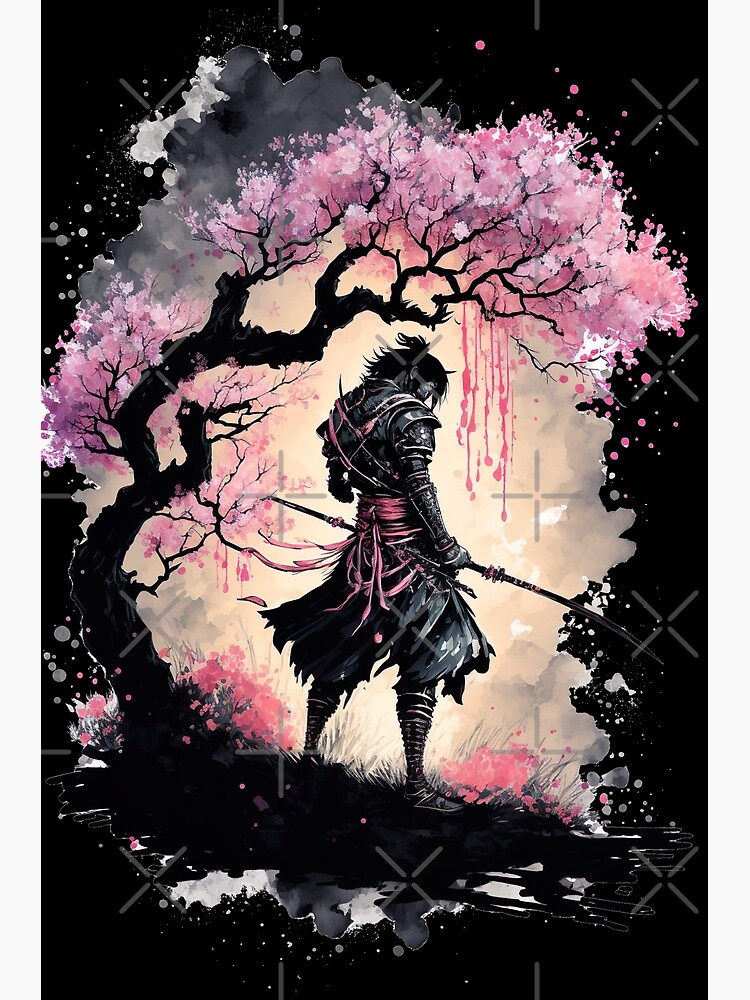This digital poster, rendered in portrait orientation, blends elements of Japanese anime and mixed-media artistry. It features a striking black background with a central splash of white, resembling paint being spilled and spread out in various directions. At the heart of this composition stands a powerful samurai, his back facing us. He holds a samurai sword in one hand while another rests sheathed on his back. The samurai is clad in a tattered black tunic and armor, with prominent black leather details and a pink sash wrapped around his waist and chest. His black hair is tied into a small ponytail, and he wears large boots. 

The samurai stands on a grassy hill dotted with pink flowers, anchored to his left by a gracefully arching cherry blossom tree. The tree's black trunk reaches over him, adorned with delicate pink blossoms that appear to drip in a watercolor fashion. Throughout the poster, light gray X's and plus signs are scattered, adding texture and complexity. Pink splatters mimic paint drips, integrating seamlessly with the samurai's surroundings and enhancing the mixed-media feel of the artwork.